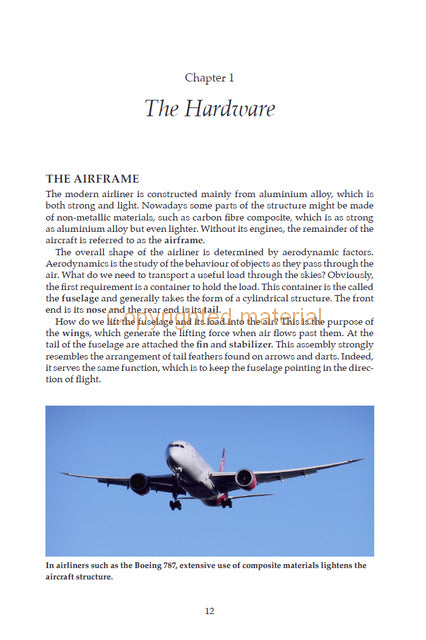The image depicts a page from a book, titled "Chapter 1: The Hardware," with a subheading "The Airframe." The text is organized into three lengthy paragraphs, discussing the construction of modern airliners. It highlights that the airframe, excluding the engines, is primarily made from aluminum alloy, known for its strength and lightweight properties. Additionally, it mentions the increasing use of non-metallic materials like carbon fiber composites, which offer comparable strength to aluminum alloy but are even lighter. This emphasis on lightweight, strong materials is crucial for aircraft like the Boeing 787, which extensively uses composite materials to reduce its overall weight. At the bottom of the text, there is a photograph of a white jet with its wheels down, presumably in mid-flight. A byline beneath the image reiterates the use of composite materials in airliners. The page also features a "copyrighted material" stamp at the base of the third paragraph.